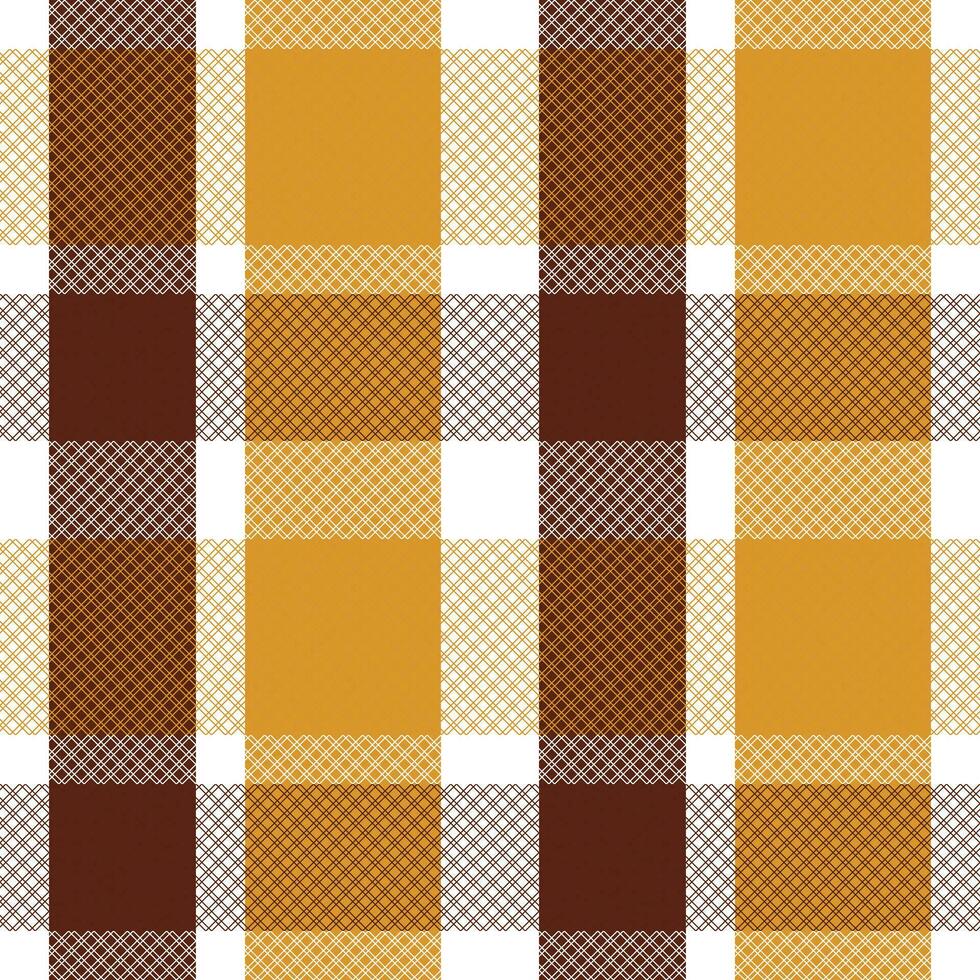This square image depicts a plastic tablecloth adorned with a detailed plaid pattern. The design features vertical and horizontal stripes creating an intricate grid. The vertical stripes alternate between a dark brown and a wider golden brown, each sequence repeating once. These intersect with horizontal stripes that follow the same color scheme: a golden stripe, a darker brown stripe, a wider gold stripe, and another darker brown stripe, with white stripes interspersed throughout. The overall effect is a harmonious plaid with brownish hues, accented by the intriguing texture of diagonal series of little dots. The combination of these elements gives the fabric a rich, textured appearance, with the colors blending into a visually appealing pattern that is both structured and intricate.